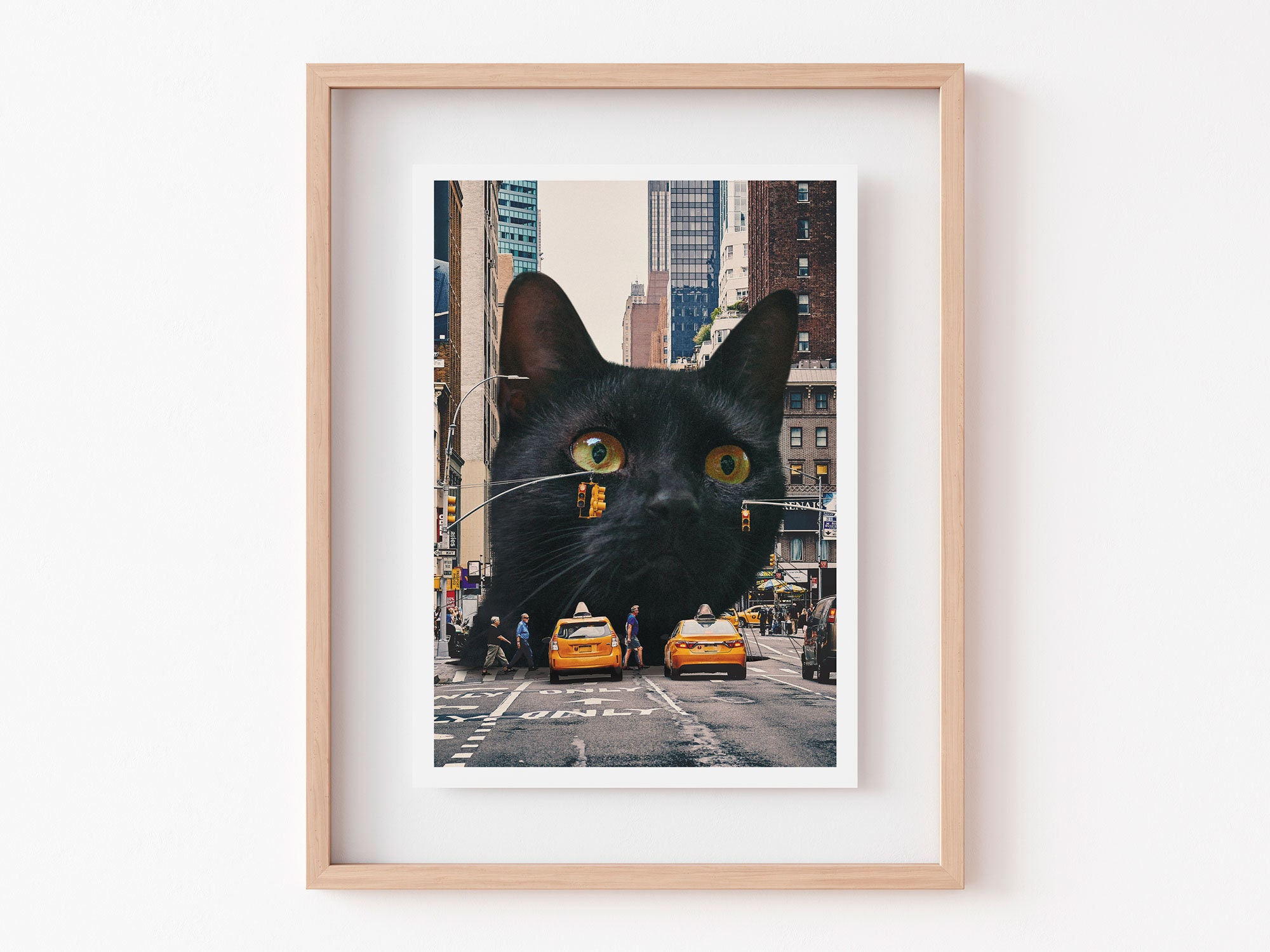This framed photograph on a blank white wall displays a surreal urban scene, presumably set in New York City, as indicated by the recognizable yellow taxi cabs. Dominating the center of the image is a gigantic, photoshopped head of a black cat, its eyes a striking mix of yellow and gold, and its expression appears somewhat distraught as it stares off into the distance. The scene is bustling yet frozen, with several pedestrians cautiously crossing the street in front of the colossal feline, and traffic halted around it, including two yellow taxis and an SUV. The backdrop reveals muted tones of brown and blue, with towering skyscrapers reaching into a white sky. Adding to the tableau's intrigue, an asphalt arrow points forward, accompanied by the single word "only." The photograph, bordered by a thick white mat and encased in a light-colored wooden frame, evokes a sense of wonder and whimsy amid the everyday hustle and bustle of city life.